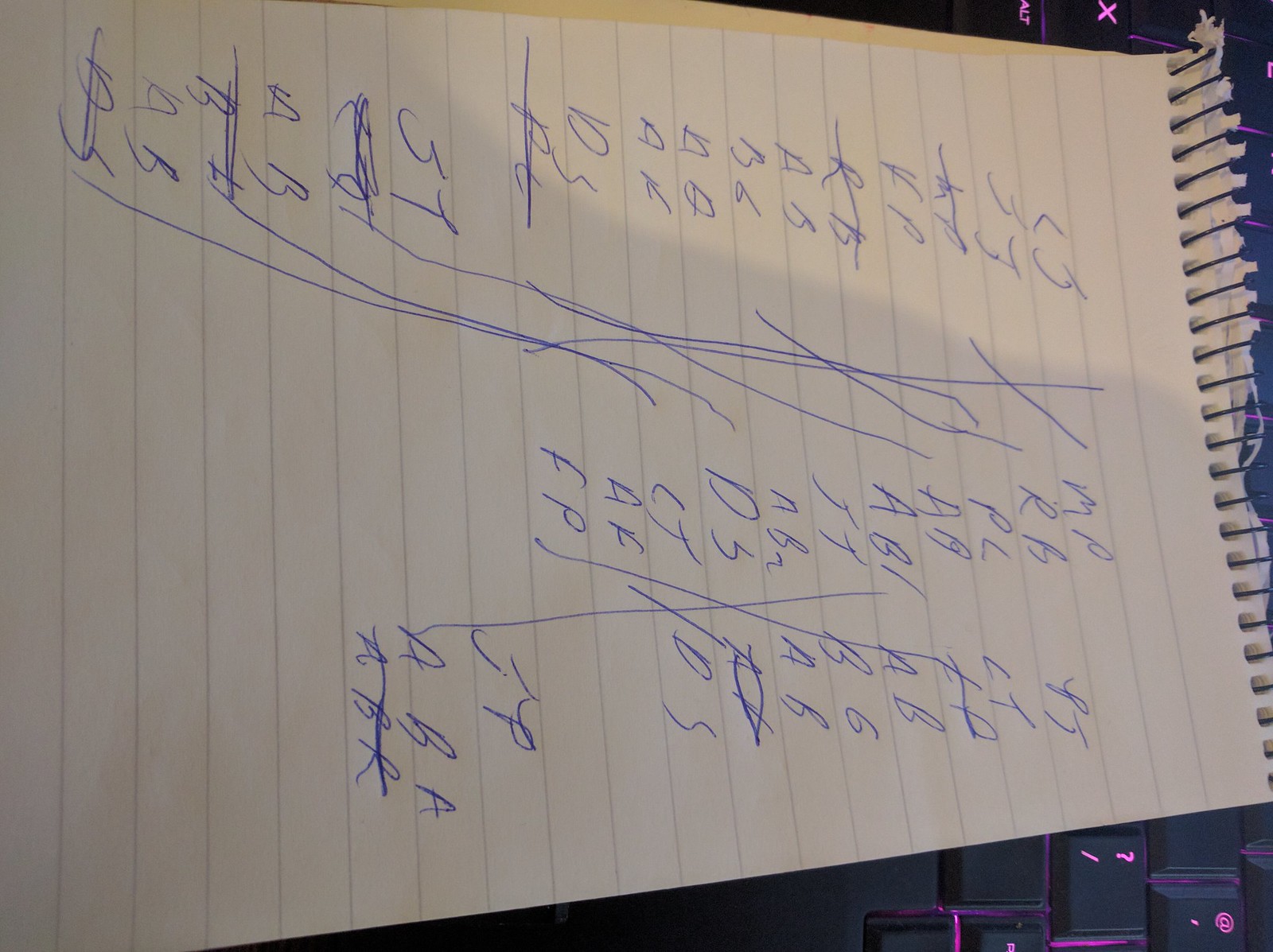In this image, which is approximately 20% wider than it is tall, a vertically-oriented notepad is prominently featured along the right edge. The notepad is topped with a black spiral binding, and several pages have been torn off. The notepad's pages are pre-printed with horizontal gray lines, typical of such stationery. The note appears to be written in blue ink and seems to be a record of scores or a list, although the purpose is not entirely clear due to the barely legible handwriting.

The handwritten content is arranged in three columns of paired letters and numbers. The leftmost column, running down the side of the page, includes entries like "SJ" at the top and "B6" as the eighth entry. A makeshift border comprised of various hastily drawn lines separates these columns. The middle column extends about halfway down the page, while the rightmost column is slightly shorter.

Adding an additional layer to the scene, the background reveals the upper part of a black keyboard, possibly that of a laptop. The keys are backlit with pink lighting, adding a distinctive and colorful element to the otherwise mundane setting.